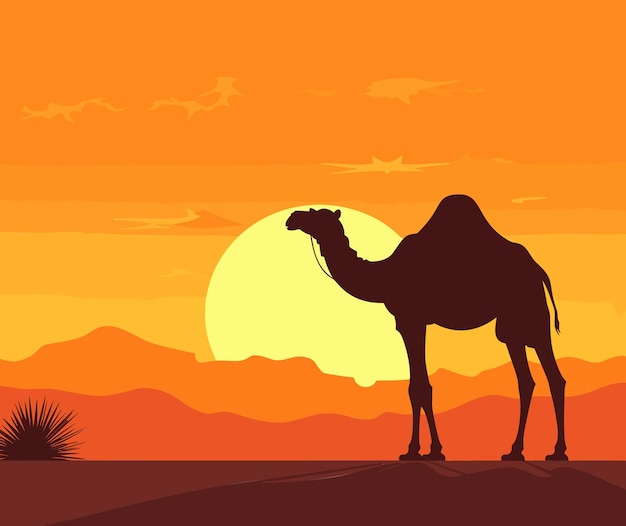In this vibrant, graphic illustration, a lone camel stands gracefully in the desert foreground at sunset. The landscape, bathed in shades of orange and yellow, reflects the warmth of the setting sun. The sky transitions from deep orange to a lighter yellow-orange near the horizon, with splotches of light orange representing clouds. Central to the composition is a pale yellow sun, casting a glow that accentuates the silhouette of the camel.

The camel, depicted in dark shadow, stands on flat, brown terrain, its single hump and possible saddle subtly defined against the bright backdrop. A spiky desert plant, also silhouetted, sits to the left of the image. Below the setting sun, layers of orange and red-orange sand dunes create depth and dimension, enhancing the scene's desert ambiance. The camel's shadow stretches forward, adding to the visual storytelling of this tranquil and stylized desert evening.